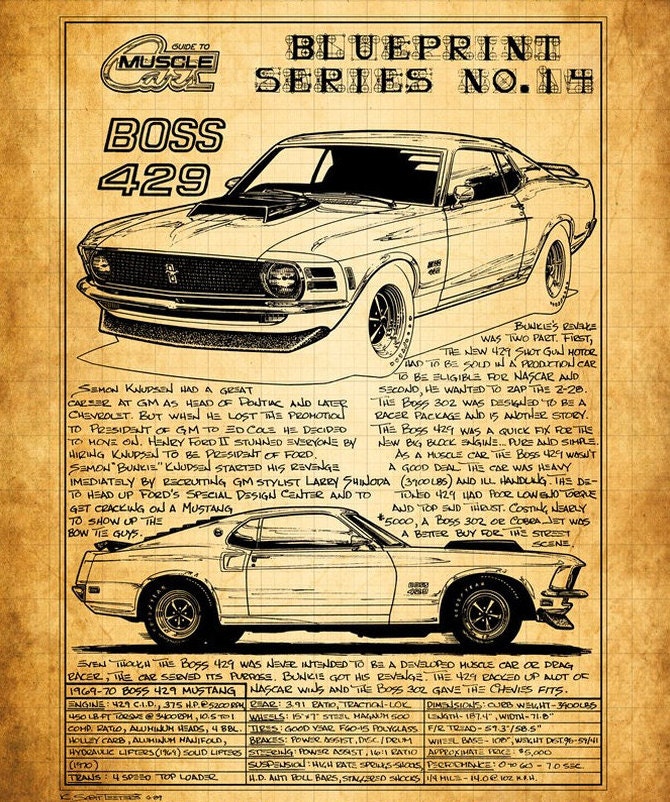This vertical poster resembles a weathered blueprint for the classic Boss 429 Mustang, part of the Blueprint Series Number 14. The parchment-colored background displays intricate, black pencil sketches of the car, presented in both front angle and side views. In the upper left corner, the heading "Guide to Muscle Cars" is prominently visible, while "Blueprint Series Number 14" and "Boss 429" are centered below.

The sketches offer a detailed view of the car, revealing its characteristic two-door, two-seater design with thick-rimmed tires. Notably, there is a vented box on the roof. Text accompanying the images narrates the significant history behind this iconic vehicle. Seaman Knudsen's career at GM and his subsequent move to Ford, where he collaborated with stylist Larry Shinoda, are highlighted. Their efforts produced the Boss 429 to fulfill NASCAR requirements and challenge competitors.

Beneath the images and historical account, the poster provides key stats and specific details about the 1969-1970 Boss 429 Mustang. While its heavy weight of 3,700 pounds and suboptimal torque are noted, the Boss 429 stands as a prime example of muscle car legacy despite its high cost and design critiques.